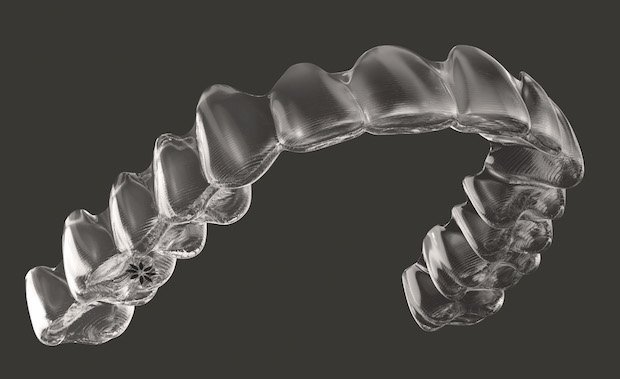This black and white image showcases a clear plastic Invisalign retainer designed for the upper teeth, prominently set against a dark gray background. The retainer, which fits over approximately 14 teeth, is displayed from an up-angle view, accentuating the bottom contours of most teeth and providing a textured, dimensional effect that visually underscores its fit. The light source, coming from the left, beautifully highlights the details, including a distinct, star or flower-shaped watermark on the second tooth from the back on the left side. The artistic rendering, reminiscent of an x-ray photograph, exhibits the retainer in shades of gray and white, creating a visually striking and realistic portrayal.